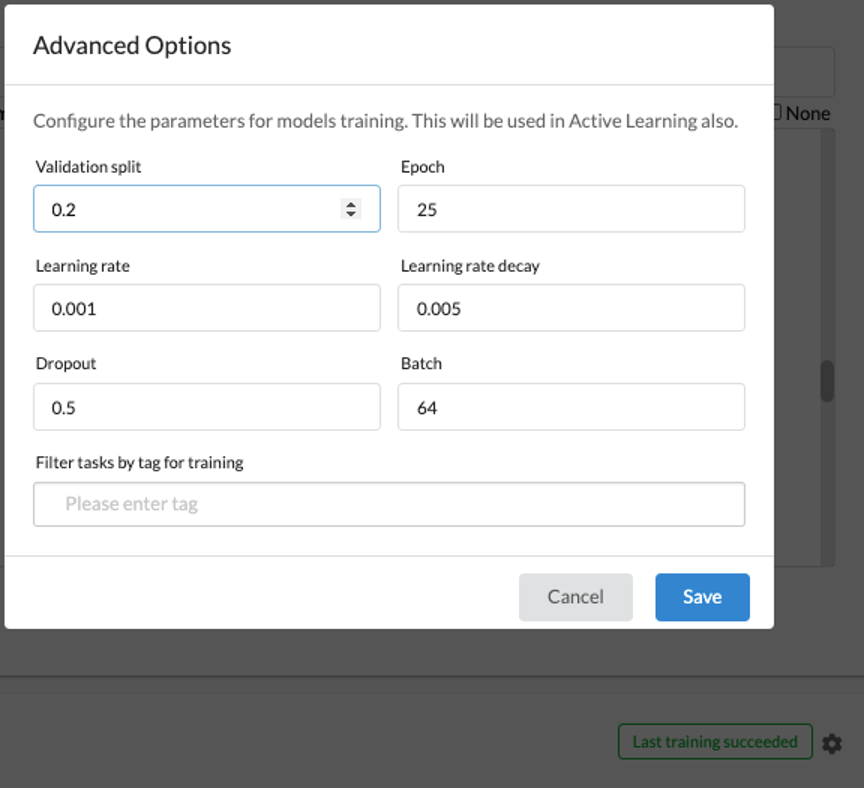This image is a detailed segment from a website showcasing advanced options for configuring model training parameters, utilized in active learning. The background is predominantly white, with the advanced options panel occupying approximately three-fourths of the entire page. Despite the prominence of the advanced options, a scroll bar is visible on the very right side, indicating additional content can be accessed by scrolling. In the bottom right, there is a gray box with the text “Last training succeeded.”

The advanced options panel includes several configuration settings spread across multiple rows:
- **Validation Split:** Set at 0.02
- **Epochs:** Set at 25
- **Learning Rate:** 0.001
- **Learning Rate Decay:** 0.005
- **Dropout:** 0.05
- **Batch Size:** 6.4
- **Filter Task Tags for Training:** A prompt to "Please enter a tag"

At the bottom of the panel, there are buttons for "Cancel" and "Save" actions. This setup allows users to fine-tune the model training parameters with precision.